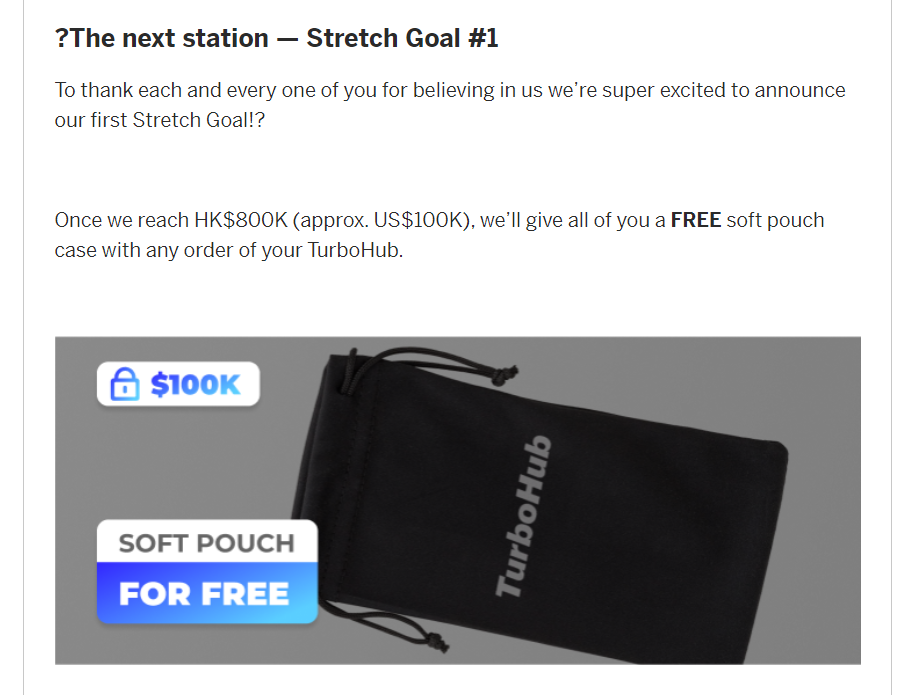This detailed caption description would fit well:

---

**Screenshot of a Webpage Section**

The image is a screenshot featuring a section of a webpage with a clean, white background and two thin vertical borders on either side. At the top, there is a text header in black that begins with a question mark and reads, "The Next Station - Stretch Goal #1." Directly below, in smaller black text, the article expresses gratitude: "To thank each and every one of you for believing in us, we're super excited to announce our first stretch goal."

The announcement continues, explaining that when the funding target of 800,000 HKD (approximately $100,000) is met, all supporters will receive a complimentary soft pouch case for any Turbo Hub order. Notably, the word "FREE" is capitalized and bolded to emphasize the offer.

Below the text is an image insert showing a sleek, black pouch with two drawstrings on either side, emblazoned with the "Turbo Hub" logo.

Additionally, there are two informational bubbles at the top left corner of the section. The first bubble features a blue lock icon against a white background, along with the text "$100,000 K." The second bubble is divided into two halves: the upper half is white and reads "Soft Pouch," while the lower half is blue and states "For Free."

---

This detailed caption describes the visual elements and the textual content clearly, providing a comprehensive understanding of the screenshot.